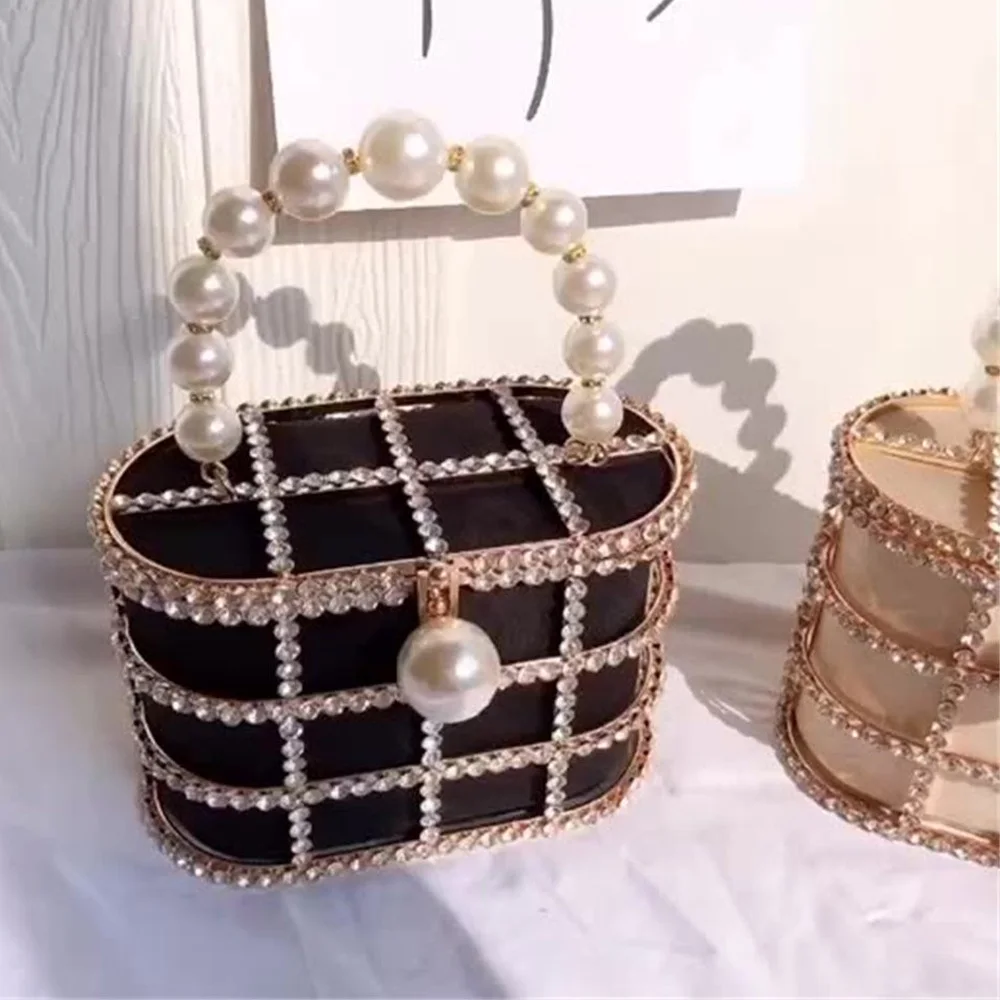The image features two elegant, box-shaped purses that resemble jewelry boxes. The primary purse in the foreground is black with a unique grid pattern created by white pearls and what appears to be diamonds arranged in a hashtag configuration. This purse has an oval-shaped top and a thicker bottom. It is adorned with a white pearl handle, which casts a shadow on the white wood wall behind it. There is a central pearl above the lock on the front of the purse.

To the right, partially visible, is another purse of the same design, but in a light pink or beige color. Both purses are set on a white tablecloth, which is only fully visible on the right side of the image, while the left side appears shadowed and gray. The white wood wall background also shows varying shadows, contributing to a dynamic lighting effect. Additionally, there is an object on the wall, possibly a picture, with a white background and three black lines, casting a shadow that adds to the image's depth. The overall setting is bright and clear, highlighting the refined details of the purses.